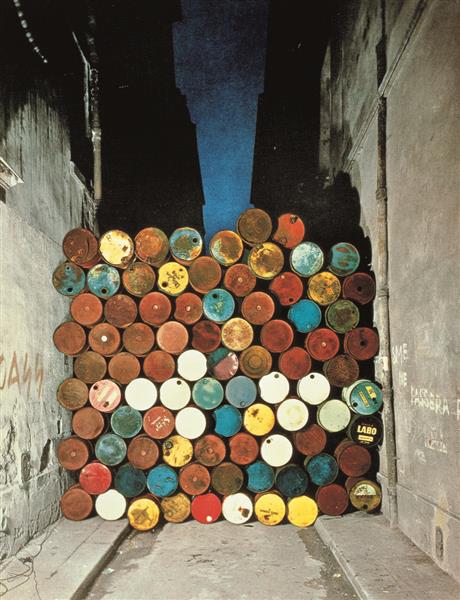In this nighttime photograph, a towering stack of metal barrels blocks an alleyway, creating a dead end. The barrels, primarily in rusty red hues but also featuring white, yellow, blue, and green, stretch approximately 12 barrels high and 13 barrels wide, filling the alley from one beige, graffiti-marked wall to the other. The vivid, spotlighted barrels stand in stark contrast to the dark sky above and the shadowy outlines of the rest of the buildings. The alley is paved, with a slightly sunken beige sidewalk running along both sides, though these are entirely obscured by the solid wall of barrels. Despite differing perspectives on the image, the dominant theme remains the extensive, multicolored assembly of metal barrels in a dilapidated urban setting.